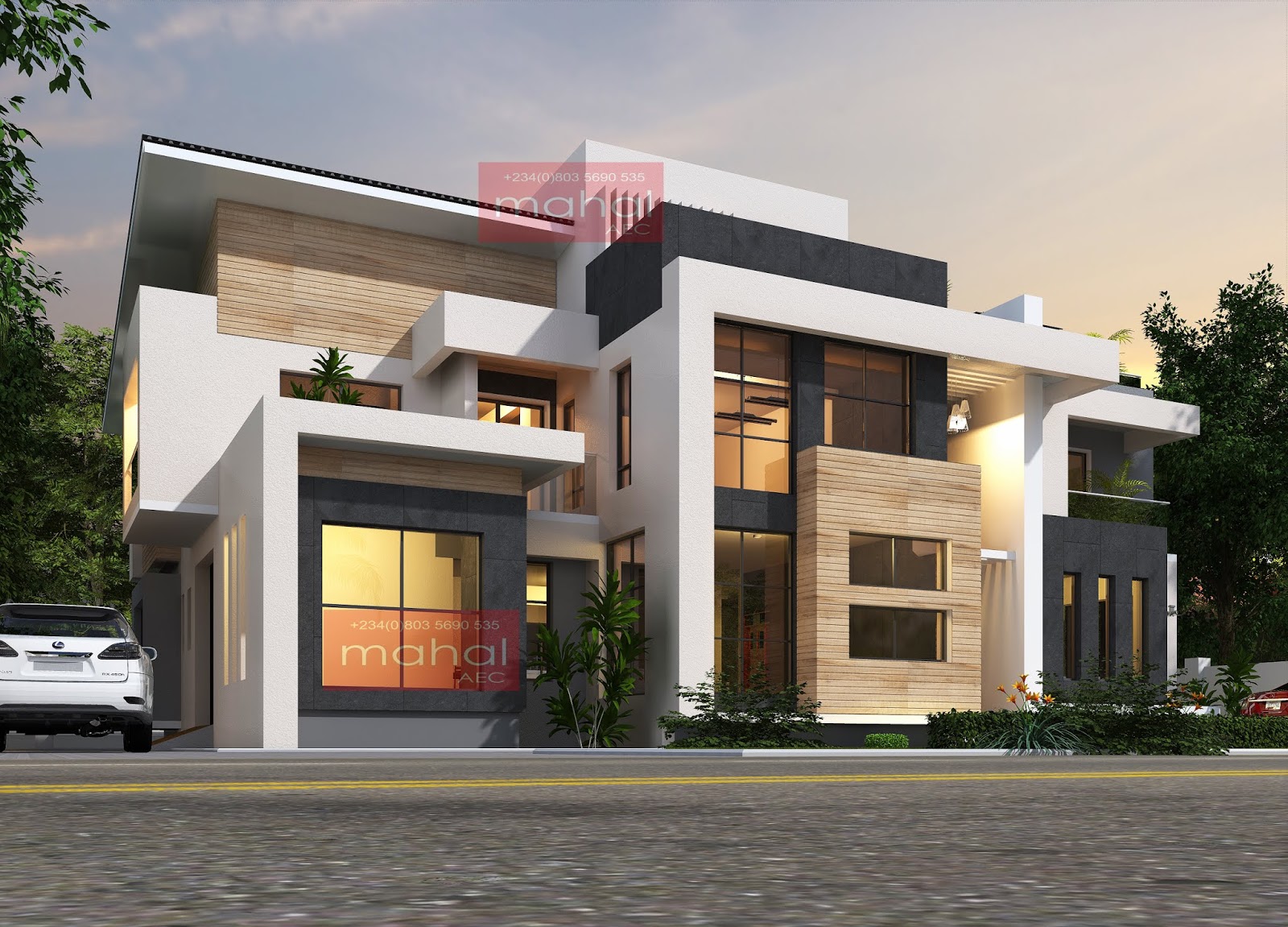The photograph depicts a modern, angular building with a strikingly contemporary design, characterized by a cubist style with large sections of black, white, and wood-paneled walls interspersed with some brown brick-like structures. The front facade features extensive glass windows and angular elements, lending the building an artistic flair. A silver Lexus is parked in the driveway to the left of the building. A sign that reads "MAHAL" is visible, suggesting a possible association with a real estate agency or another business. The street in front of the building resembles a main thoroughfare rather than a suburban street. The image captures a misty sky, imbued with gray and blue hues, indicating either dawn or dusk, while lush, green trees on the left suggest a spring or summer setting. Some bushes are situated in front of the building, enhancing its landscaped aesthetics. The overall composition hints at the possibility of the building being either a residence or a commercial property, given its intricate and modern architectural elements.